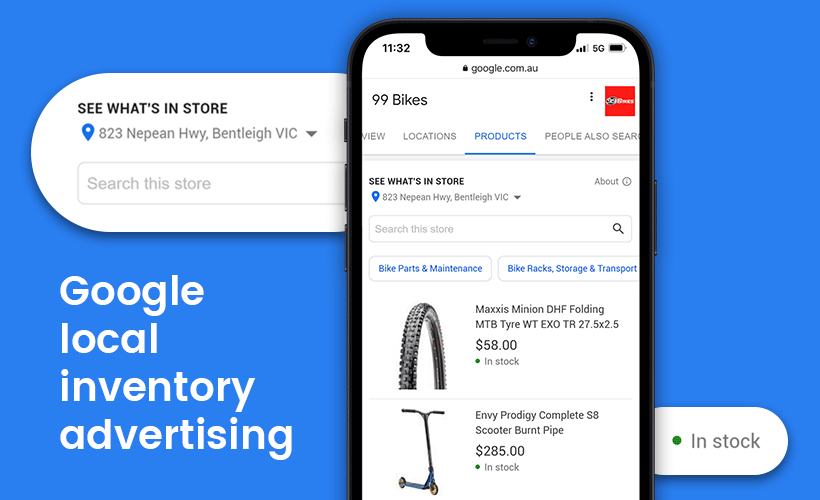The web page image is designed horizontally, featuring a blue background. Prominently positioned on the lower left-hand side is bold white text stating, "Google Local Inventory Advertising." Above this, a white speech bubble contains the text, "See what's in store," accompanied by a location icon. Within a dropdown menu, the address "823 Nippan Highway, Bentley VIC" is displayed, along with a button labeled "Search this store."

Overlaying the right side of this upper text box is an image of a smartphone, showing a search results page for "99 Bikes." The phone's display has a white background, with the header bar highlighting "Products" in blue and underlined. Below the header, there is a search box and two buttons: "Bike Parts and Maintenance" and "Bike Racks Storage and Transport."

Displayed beneath these buttons are two illustrated products. The first product is a "Maxxis Minion DHF Folding MTB Tire WTEXOTR 27.5 x 2.5," priced at $58. The second product is an "Enve Prodigy Complete S8 Scooter Burnt Pipe," priced at $285. Both items are marked as in stock. Adjacent to the smartphone image, at the lower right-hand corner, there is a small white bubble with a green circle indicating that the items are "In stock."